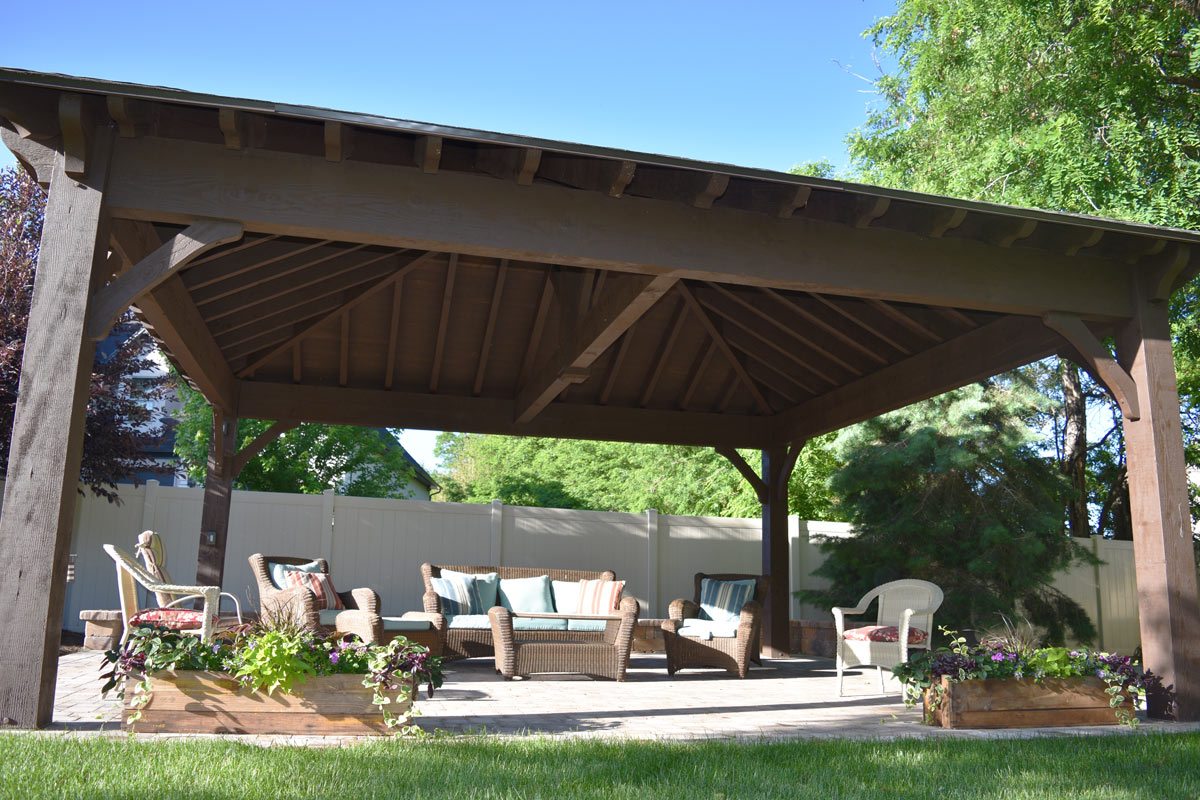This backyard oasis features an inviting patio area situated on a large, whitish stone or cement slab and covered by a flat-roofed gazebo with brown wooden posts. Beneath the shelter, there is a set of wicker patio furniture, including a three-seat wicker sofa, single wicker chairs, and a wicker coffee table. Wooden planters brimming with purple flowers and green foliage flank the patio, adding bursts of color to the scene. The foreground is dominated by lush green grass, extending around the patio, while the background showcases a tall, white cement wall. To the left, a house is partially visible, and to the right, large trees provide additional shade and a sense of seclusion. The setup suggests a perfect spot for relaxation and social gatherings.